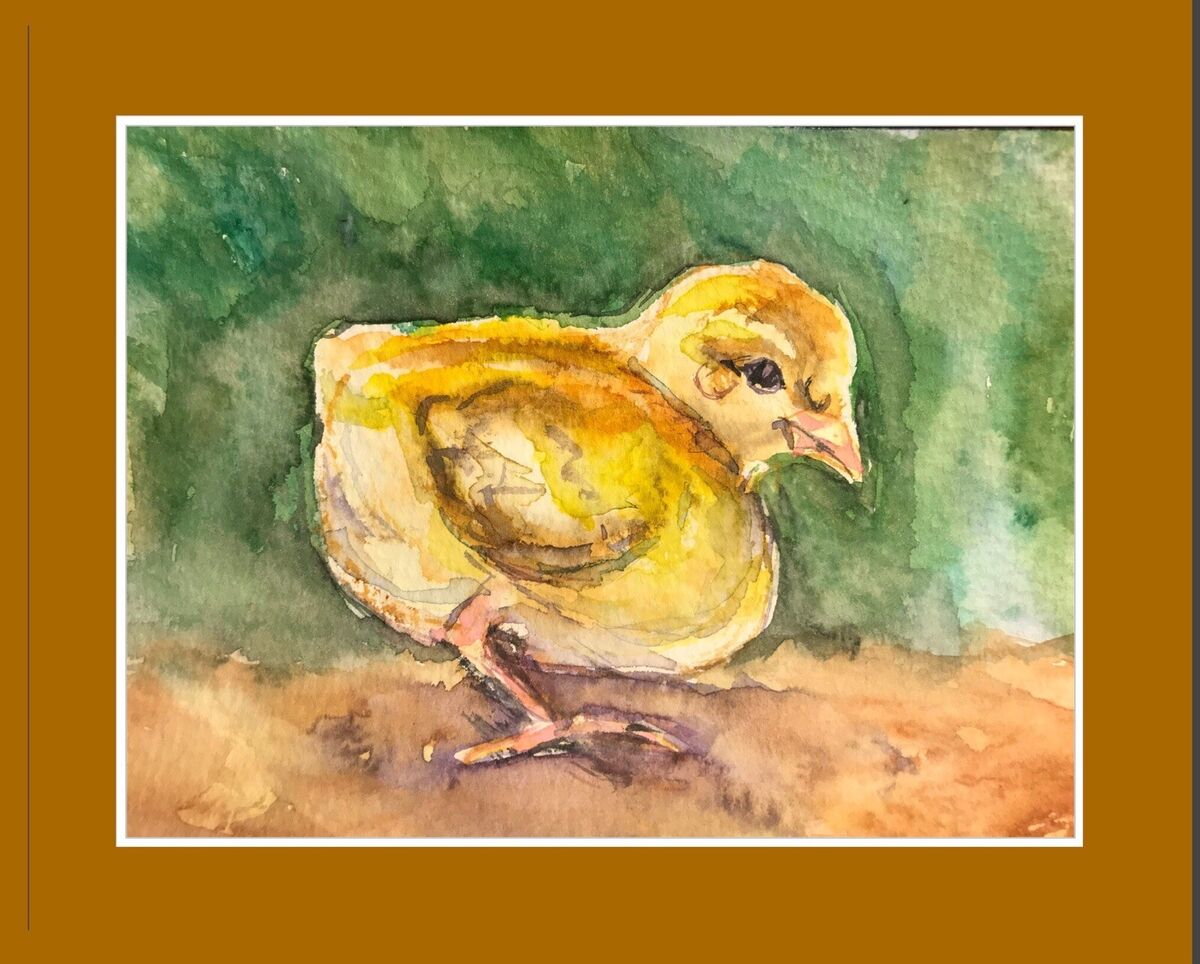This image showcases a detailed watercolor painting of a small, round-bodied baby chick, prominently featured and centered within a square poster painting. The chick is rendered in vibrant yellows, with orange wings, a small orange beak, and lightly colored orange legs. The painting is bordered by a dark tan matte, with an additional thin white border that frames the artwork.

The chick is seen in profile, with its right side facing the viewer, giving a clear view of only one slightly bent leg. The background is a mixed palette of greens, with dark and light green tones blending into light white and blue hues, suggesting an outdoor setting, potentially a meadow. The ground upon which the chick stands is depicted in tones of light brown and orange, with a clayish, dirt-like appearance. Despite the simplicity of the watercolor style, the vivid colors and the zoomed-in composition make the chick the focal point of this charming and lively painting.